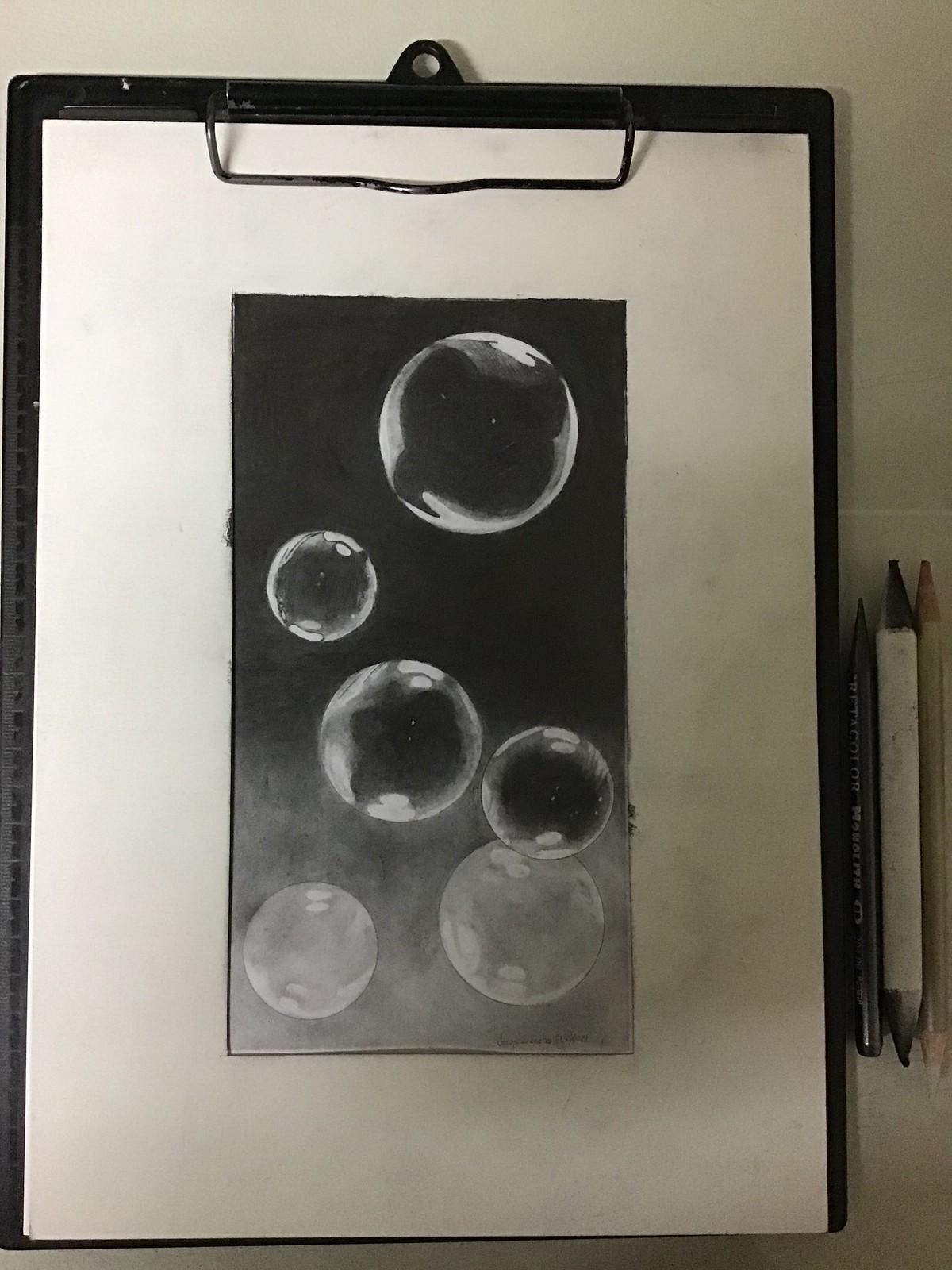This black-and-white image features a detailed drawing of six bubbles, each outlined in white and shaded to create a 3D, realistic appearance. The bubbles are predominantly black on the inside, gradually lightening in areas, with two particularly light gray ones at the bottom. They are set against a darker background at the top that transitions to gray toward the bottom, giving the impression that the bubbles are floating in air.

The artwork appears to be created using a combination of markers, pencils, and possibly charcoal, evidenced by the smeared charcoal marks on the white matting around the drawing and beyond the vertical picture area itself.

The image is centered on a white piece of paper clipped to a black clipboard. There are three drawing instruments laying beside it: a skinny gray pencil with white writing, a fatter white and gray pencil, and a beige one, suggesting the various tools used to create the intricate details of the bubbles.

Overall, the image showcases a mix of traditional art media to bring a simple subject to life with depth and realism.